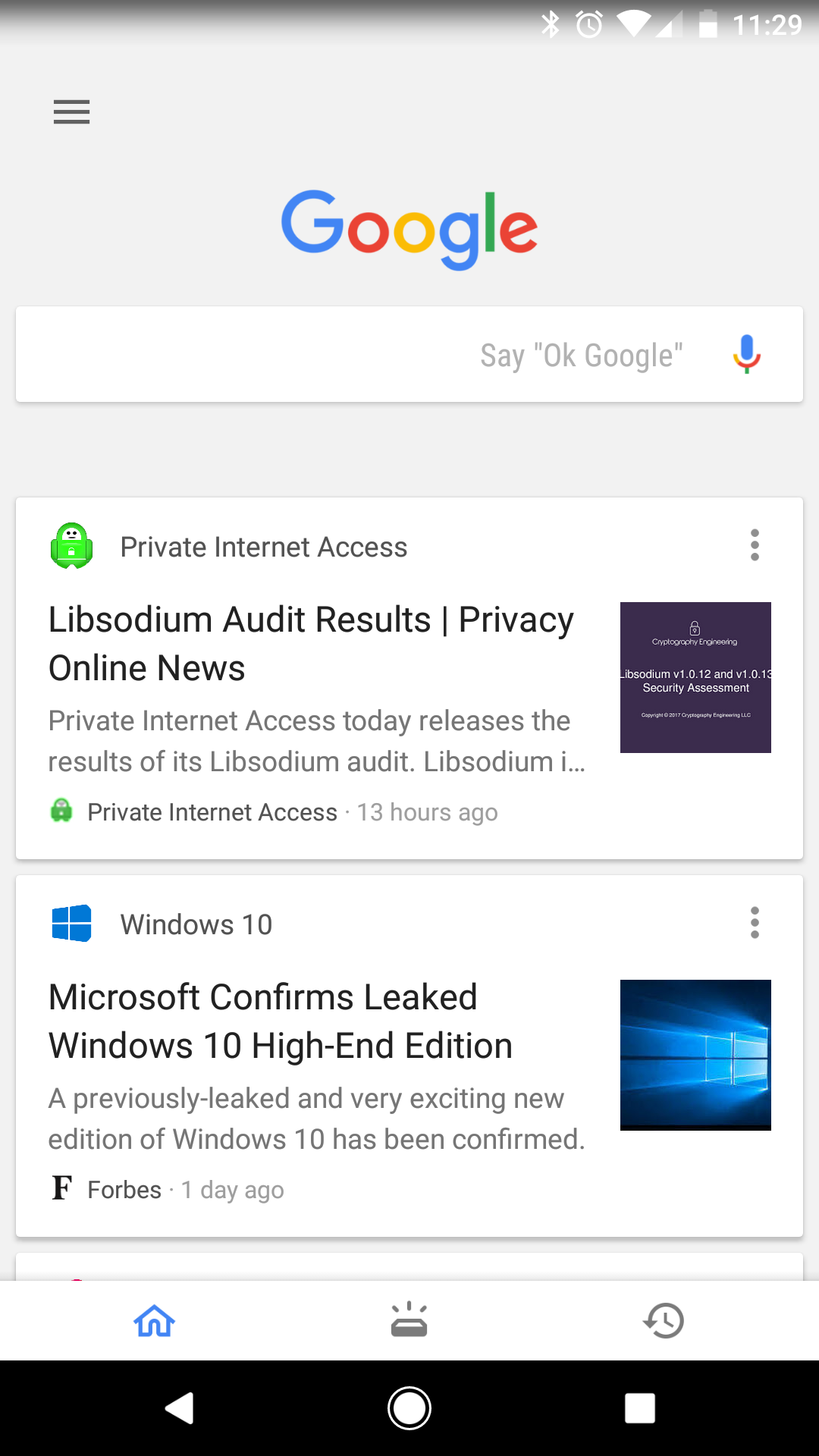This screenshot captures a Google search page interface. At the top right-hand corner, we see a series of icons symbolizing the status of various phone functions: Bluetooth, alarm, Wi-Fi, cellular reception, and battery life. The current time displayed is 11:29. Centered below these icons is the Google logo followed by the familiar Google search bar. Inside the search bar, to the right, the text reads "say 'OK, Google'," accompanied by a microphone icon, indicating a voice search option. 

Below the search bar, there are two informational blocks. The first block is titled "Private Internet Access" and features the green Android symbol. A line of text below the title reads, "Liposodium audit results / Privacy Online News." The second block below this is headlined "Windows 10" with the content below indicating, "Microsoft confirms leaked Windows 10 high-end edition."